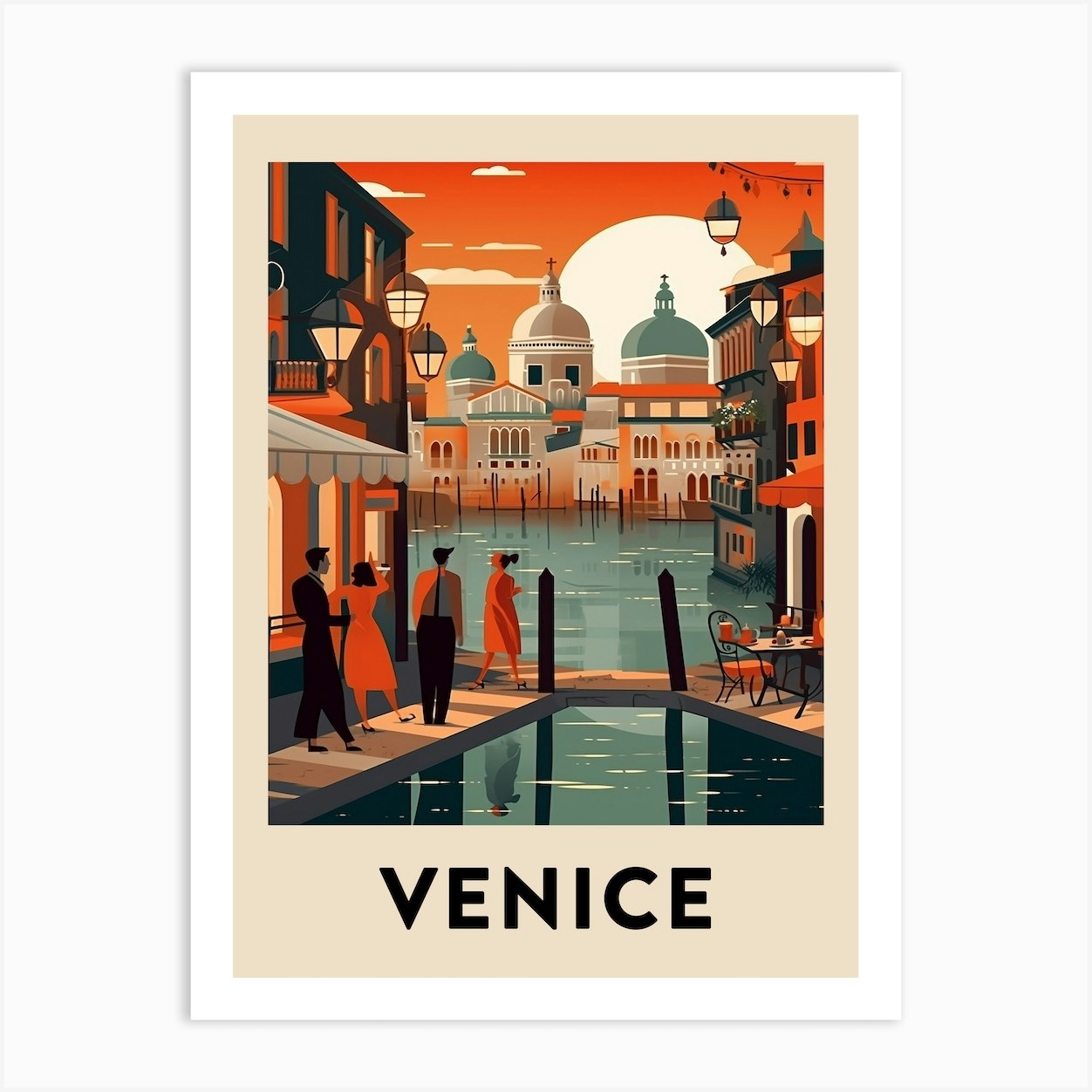This is a detailed watercolor-style artistic poster advertising Venice, Italy, framed with a white border and a tan inner border. At the bottom, in bold black letters, it says "Venice." The scene is set at sunset, with a rust-orange sky and white clouds, casting a warm glow of reds and yellows over a picturesque cityscape.

In the foreground, there’s a curving boardwalk forming a reverse U-shape, wrapping around green and gray canal waters. Several men and women, dressed in suits and dresses, walk along the boardwalk, seemingly headed to a charming bistro. On the right side of the boardwalk, a wrought iron table with two chairs sits, adorned with food and possibly coffee. 

The background showcases an array of buildings: three-story structures in dark brown hues, some with chocolate brown and tan colors, accented with green and red roofs. One of the buildings, with a cross on its dome, highlights a church. Some of the buildings feature charming awnings, flowers in the windows, and hanging street lights, enhancing the romantic Venice atmosphere.

Overall, the vibrant colors, detailed architecture, and serene canal scene perfectly capture the enchanting and timeless allure of Venice.